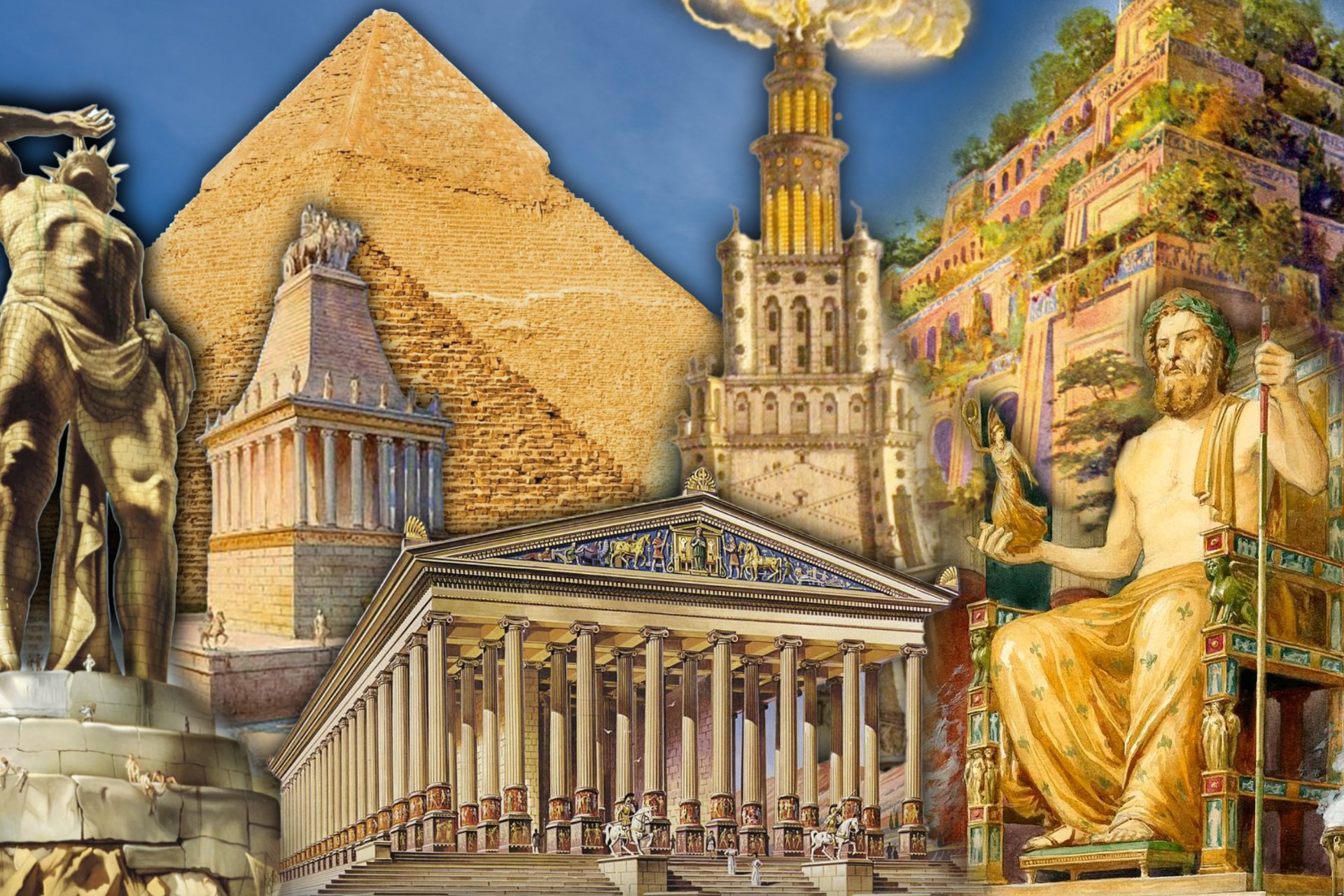The artwork appears to be a digitally created collage, blending photographs and illustrations of various ancient architectural structures and statues. In the background, a golden sandstone pyramid, likely from ancient Egypt, stands prominently against a bright blue sky. The foreground is dominated by the Parthenon, an iconic example of Greek masonry with its recognizable columns and elaborate ornamentation. On the right side, a Greek statue of a muscled, draped man commands attention, opposite a kingly figure seated on a throne, wearing a wreath and holding a staff, garbed in golden-green attire. Additionally, there’s another pyramid structure reminiscent of Mayan architecture, featuring distinct layered levels and lush greenery. The overall composition of overlapping stone edifices and sculptures from ancient civilizations, accentuated by shadow effects, creates a visually rich and intricate portrayal of humanity’s classical heritage.